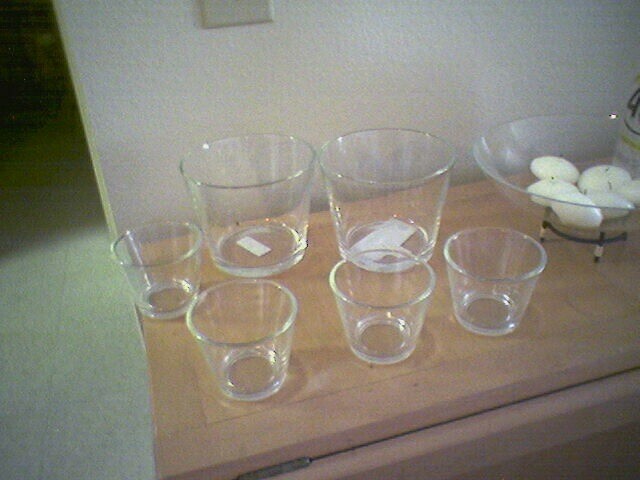This photograph, most likely taken in dim light, showcases a close-up of a wooden expandable table or shelf with visible hinges, positioned against a wall in a home. The surface, a medium to light grayish-brown color, is illuminated by light shining down onto the table and the flooring beyond it. On the table are various clear glass cups: four short, wide-flared glasses in the foreground, and two taller, larger glasses behind them, each with a white sticker on the bottom. To the right of the glasses is a clear bowl resting on a simple black metal stand, which holds six white candle-like eggs, possibly tea candles. A bottle marked with the number '4' and a light fixture on the wall add detail to the space, with a light switch and a possible hallway visible in the background.